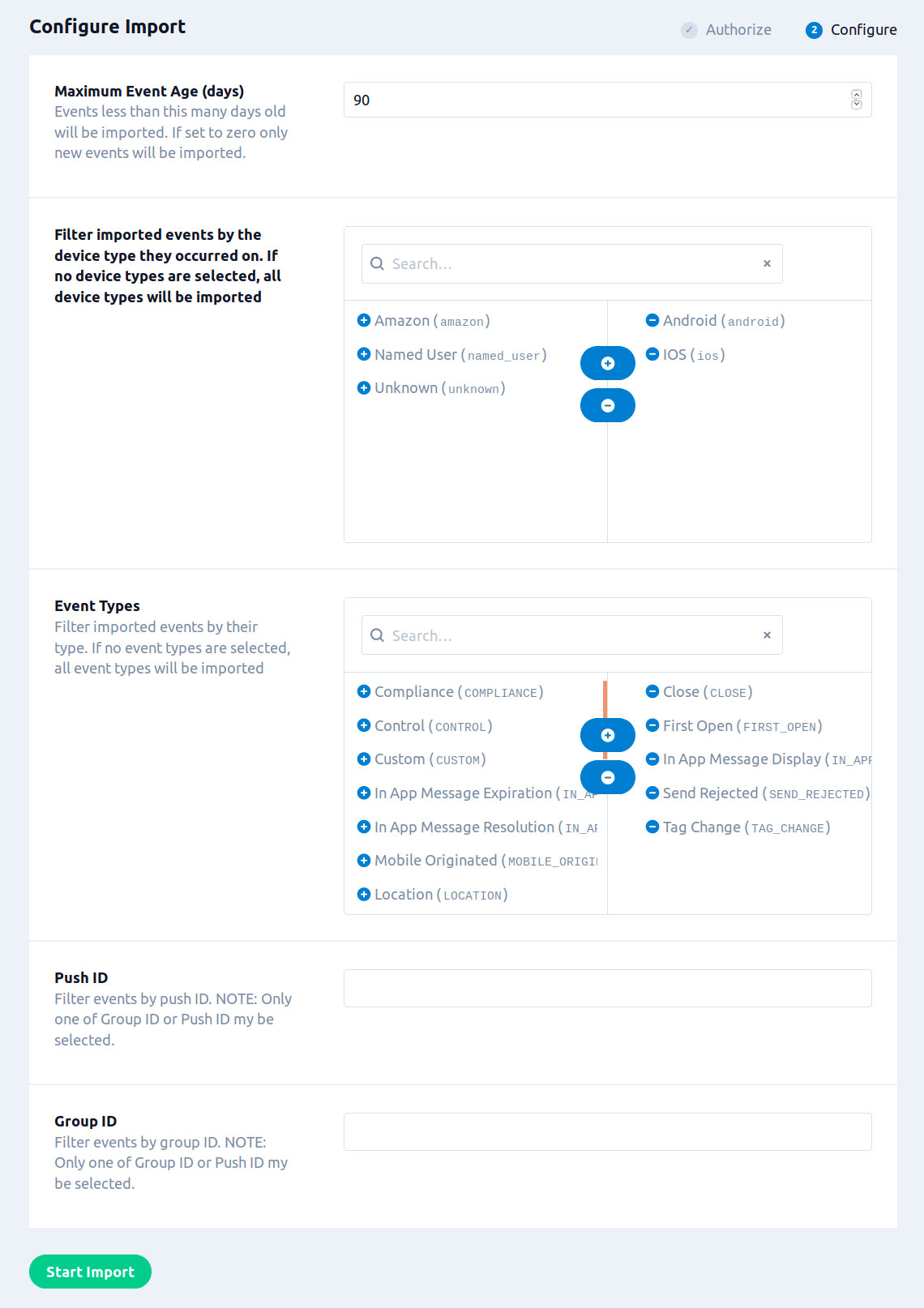**Caption:**

The screenshot showcases a filter configuration menu designed for importing events. The interface features a sleek blue border surrounding a white interior. At the top-left corner, the menu header displays the text "Configure Import" in bold black font. To the right, options labeled "Authorize" and "Configure" are visible.

Below the header, there's a section titled "Maximum Event Age (Days)": it specifies that events must be less than a certain number of days old to be imported, with the current setting at 90 days.

Further down, the menu allows filtering of imported events by device type. If no device types are selected, all types will be imported. A search box is provided for ease of filter selection. The current filters listed are: Amazon, Named User, Unknown, Android, and iOS, each represented by blue buttons that facilitate adding or removing these options.

The next section underlines that events can also be filtered by type. Again, if no event types are chosen, all types will be imported. Another search box is available for this filter. The listed event filters include: Compliance, Control, Custom, In-App Message Expiration, In-App Message Resolution, Mobile Originated Location Close, First Open, In-App Message Display, Send Rejected, and Tag Change. Blue buttons are again provided for adding or subtracting these filter options.